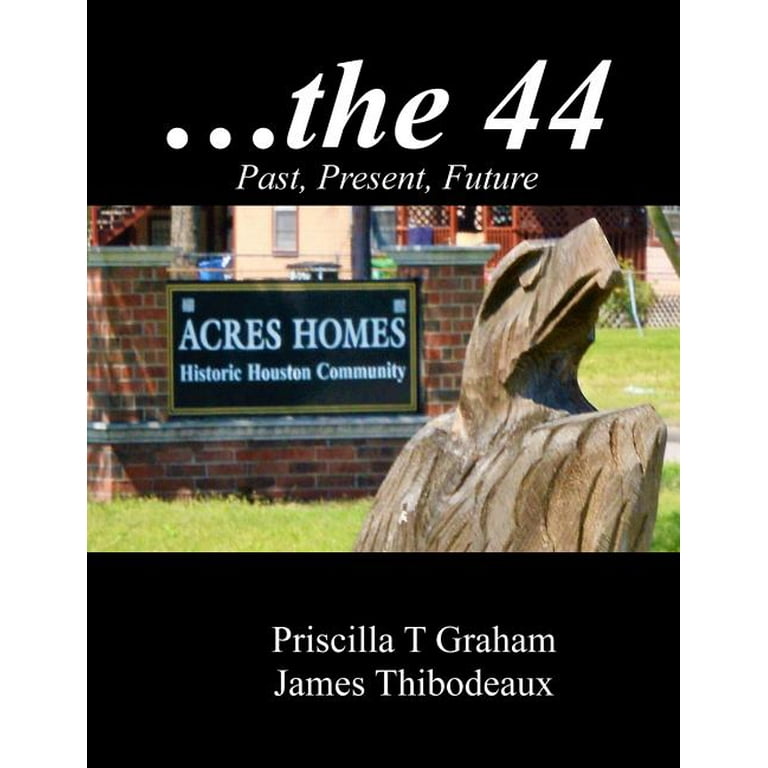This appears to be an advertisement or magazine page featuring an eye-catching title at the top which reads "...D44" in very large serif typeface, followed by the phrase "past present future" in smaller letters within a black rectangular box. Dominating the central part of the layout is a detailed image of a brick fence adorned with a black sign that boasts a gold rectangle and reverse letters proclaiming "Acres Home Historic Houston Community." The image, taken in daylight, reveals green grass enveloping the scene, and prominently in the foreground, a roughly carved eagle—likely made of wood or concrete—is visible with its head raised skyward. Additional text in a black box at the bottom credits "Priscilla T. Graham and James Thibodeau." The backdrop hints at other structures with windows and stairs, contributing to the sense of a well-lit, historical neighborhood.